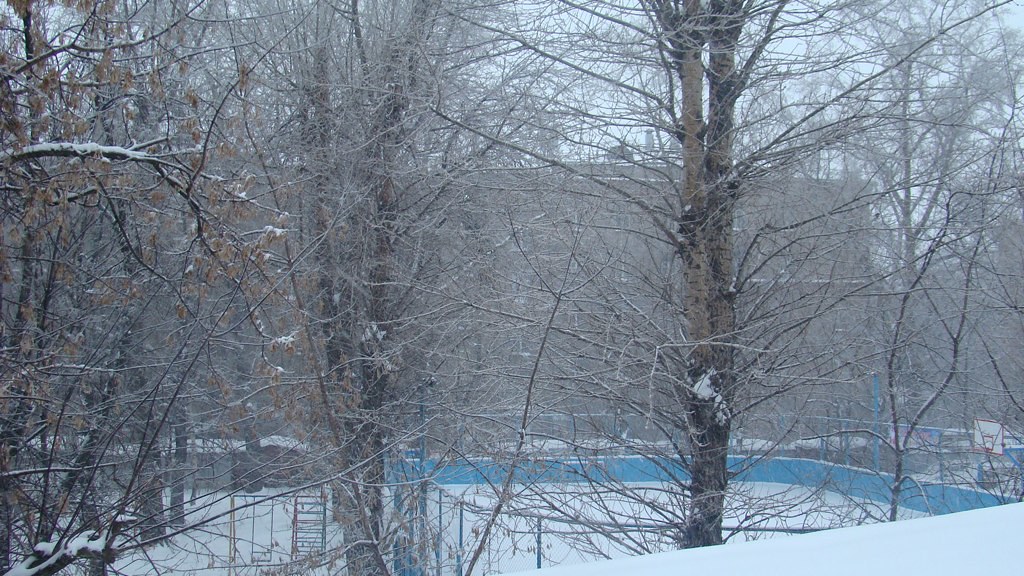The image depicts a snowy, winter day, captured outdoors under a gray sky. In the foreground, the scene is dominated by leafless trees with branches covered in snow, hinting at the cold season. The ground is completely blanketed in white, enhancing the wintry atmosphere. Toward the bottom left, a playground area is visible, featuring a swing set and a blue fence that likely encloses the space. Just beside it, a basketball hoop with a white and red backboard stands out amidst the snowy landscape.

In the background, partially obscured by the trees, there appears to be a red brick building. Also visible is an outdoor ice hockey rink, identifiable by the blue boards and chain-link fence surrounding it. The image is taken from an elevated vantage point, possibly the roof of a house, offering a comprehensive view of the snow-laden scenery. The overall feel of the photo evokes a quiet, serene winter day.